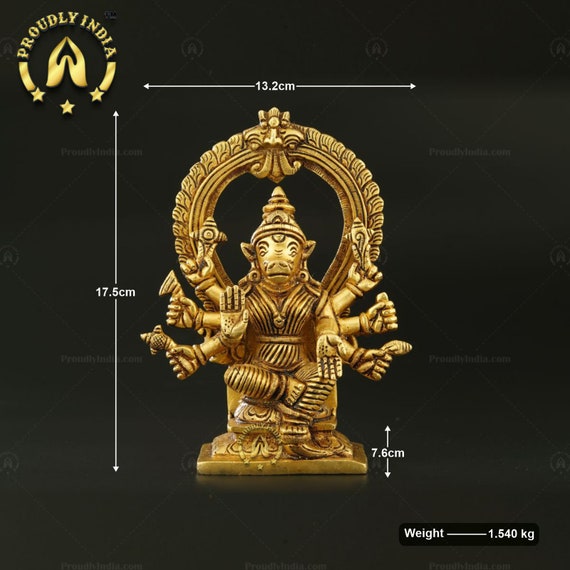The image features a golden Indian statue, prominently marked in the top left corner with a gold logo and the inscription "Proudly India." The statue, which stands 17.5 centimeters tall and 13.2 centimeters wide, sits on a pedestal measuring 7.6 centimeters across. It weighs 1.540 kilograms. The deity depicted is a hybrid of human and animal traits, often associated with Indian mythology. This figure has six arms, with each hand holding various objects, and its legs are arranged in a crossed position. Behind the figure is a large circular wreath. Additionally, there are two little hands forming an upside-down heart with their thumbs and fingers, accompanied by three stars.